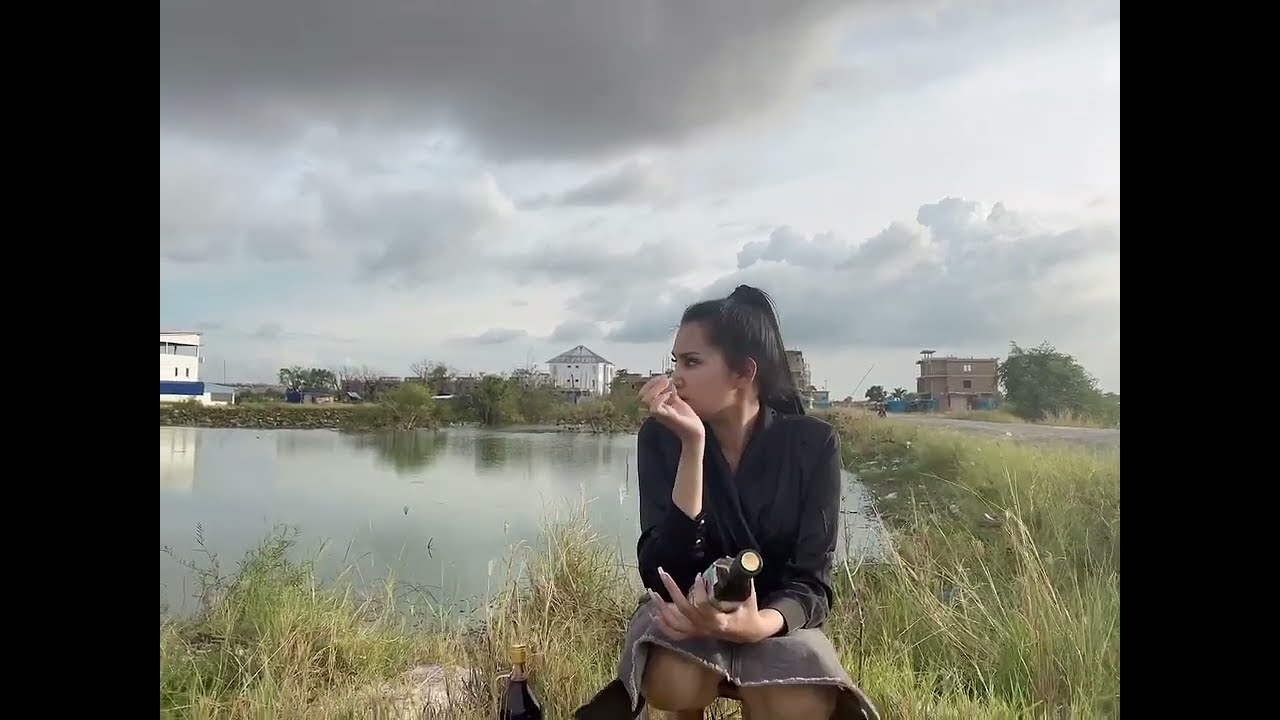In the image, there is a young girl squatting by a small lake, surrounded by greenery and an unkempt road. She is wearing a black jacket and a grey mini skirt, with her thighs and knees visible. The girl has black hair tied back and is looking sideways, not at the camera. In her left hand, she holds a bottle that looks like an alcohol bottle, and another similar bottle is placed on the ground behind her. Her long fingernails are noticeable. The background features a cloudy sky, indicating daytime with good weather. There are some houses visible in the distance, but no vehicles on the road. The scene appears to be rural or semi-urban, and the photo was taken by someone else, capturing the girl posing amidst tall bushes and the body of water.